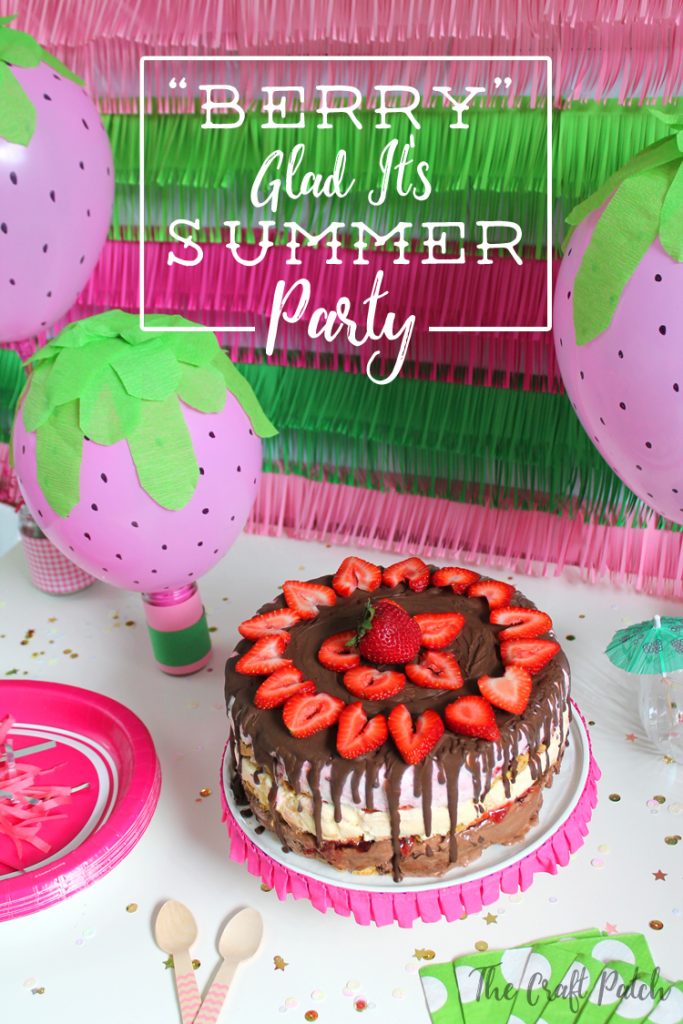The image is a vibrant, full-color promotional piece likely used as an invitation for a summer party. The overall design features both computer-generated and real elements, with a modern and girly aesthetic. Centrally, a delectable chocolate layer cake adorned with fresh strawberries and a drizzle of dark frosting sits on a white table. 

Surrounding the cake are whimsical pink balloons designed to mimic strawberries, complete with green felt leaves and black speckles. The upper center of the image contains a white rectangular box with mixed typeface text, stating "Berry" in quotes, GLAD IT'S SUMMER PARTY. The text alternates between capital letters and cursive script, amplifying the playful and stylish theme.

Additional elements include green and white polka-dot napkins, pink plates, and spoons positioned neatly around the table. In the bottom right corner, "The Craft Patch" is printed in gray cursive. The background showcases a vibrant, pink and green skirt-like decoration, enhancing the festive, summer vibe of the image.